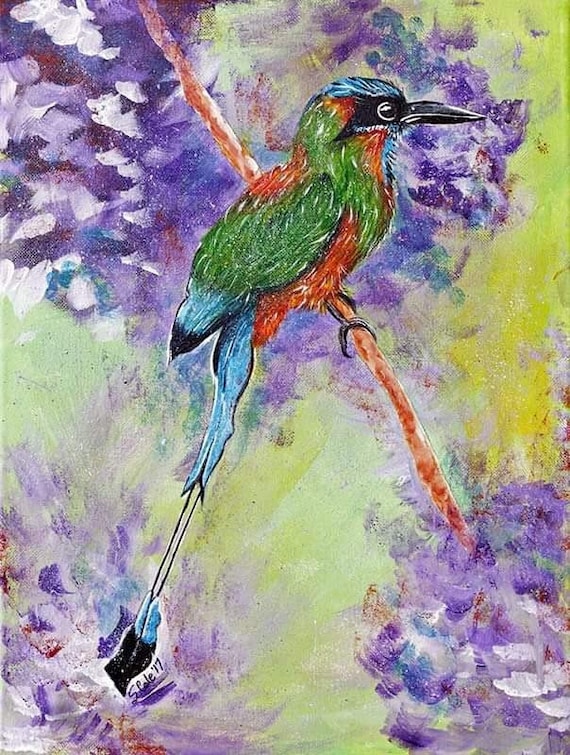This is a detailed drawing, possibly a painting, of a vibrant bird perched on a diagonal brown branch that stretches from the top left to the bottom right of the vertical rectangular frame. The bird is facing to the left and is slightly above the center of the image. Its head is blue with black markings around its eye and a long, curved black beak that tapers to a point. The bird's back and wings are predominantly green, with blue tips and black at the ends. Its breast is bright orange, transitioning to green in the belly area and again to orange. The bird features a strikingly long tail that is light blue with a black tip, from which extends what appears to be a thin, bone-like protrusion down to a small black segment, resembling a flag.

The background is rich and varied. The upper left is filled with purple and white brush strokes, with similar textures in the upper and bottom right corners. There are purple and white splashes around the bird, possibly indicating abstract flowers. The bottom left has more purple coloring mixed with some red. The upper right corner is marked by a yellow area that transitions to a light green as it moves towards the middle. The lower center part of the image appears yellowish-green. Among this colorful setting, beneath the bird's tail, is the signature "S-P-A-L-E '17."

Overall, this artwork combines a kaleidoscope of colors, bringing to life a beautifully detailed and exotic bird against a dynamic and textured background.